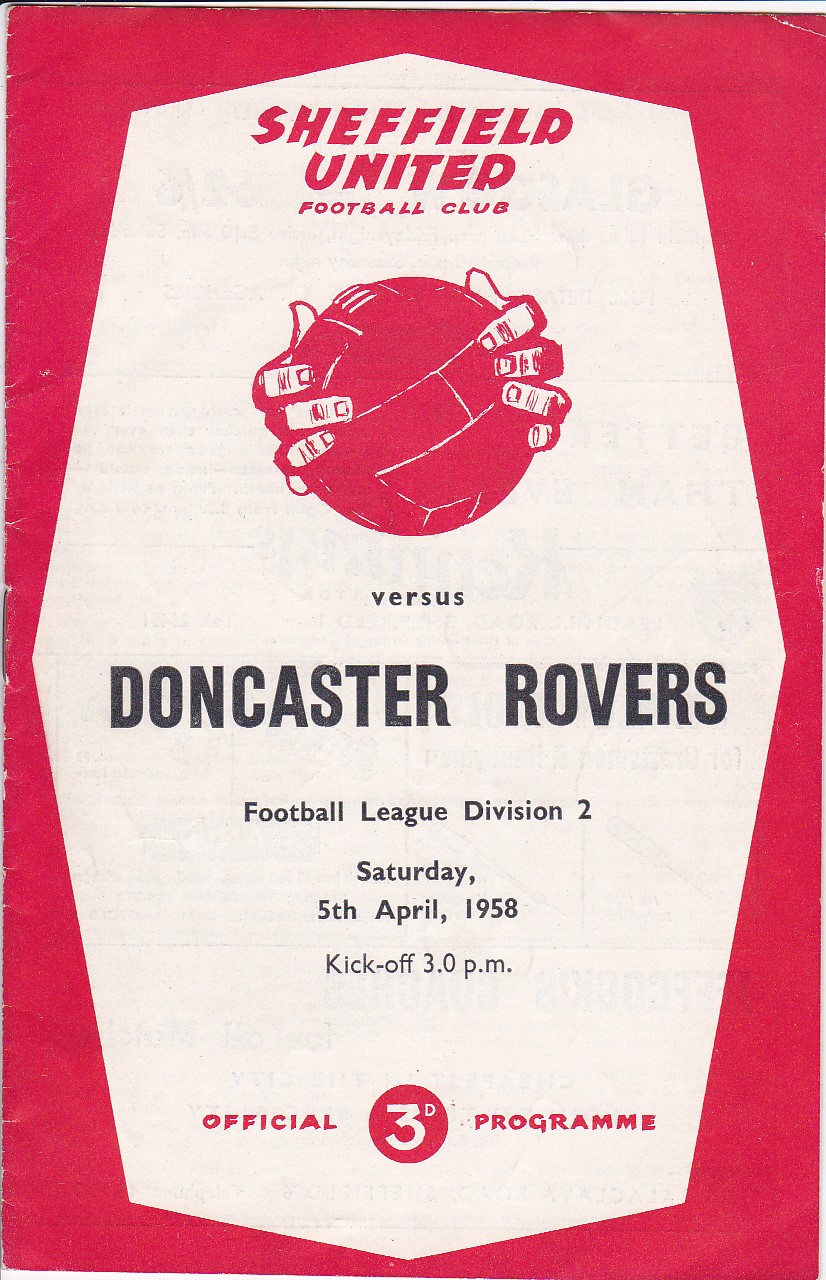This image is an official program for a Sheffield United versus Doncaster Rovers football match, dated Saturday 5th April 1958, with a kickoff at 3.0 p.m. The design is distinctly 1950s, featuring three colors: black, white, and red. The central graphic element is an elongated octagon, oriented on its points, with a red border and a white background. The top of the octagon displays "Sheffield United Football Club" in red text, indicating Sheffield United as the home team. Below this is the club’s logo, a red ball with hands. Following are details of the match: "versus Doncaster Rovers" in black text, accompanied by information about the Football League Division 2 fixture. The bottom of the program features "official program" in red text, with a circular red emblem in the center that contains white text reading "3D." The edges of the program are highlighted with a red outline, enhancing its vintage aesthetic.